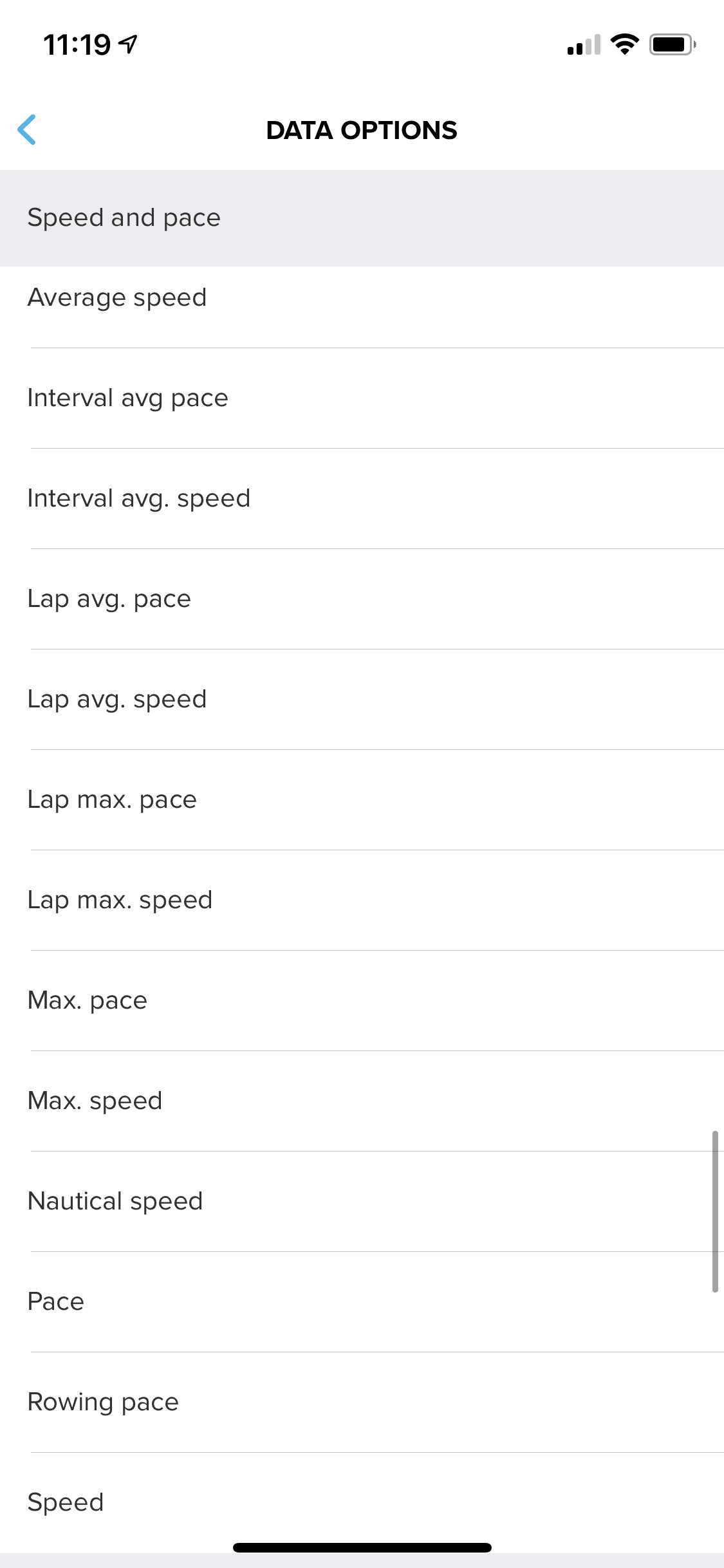The image displays a settings screen titled "Data Options," showcasing an extensive list of various speed and pace measurements. The list includes categories such as speed, pace, average speed, interval average pace, interval average speed, lap average pace, and lap average speed, all primarily focused on tracking different forms of movement over time and distance. Additionally, the list features more specialized measurements like nautical speed and rowing pace, suggesting the app is versatile and not limited to running. The screen has a clean design with a white background and black text, and there's a navigation option to go back. The notification bar at the top is also visible. Users can scroll up or down to access even more measurement options that extend beyond the visible portion of the screen.